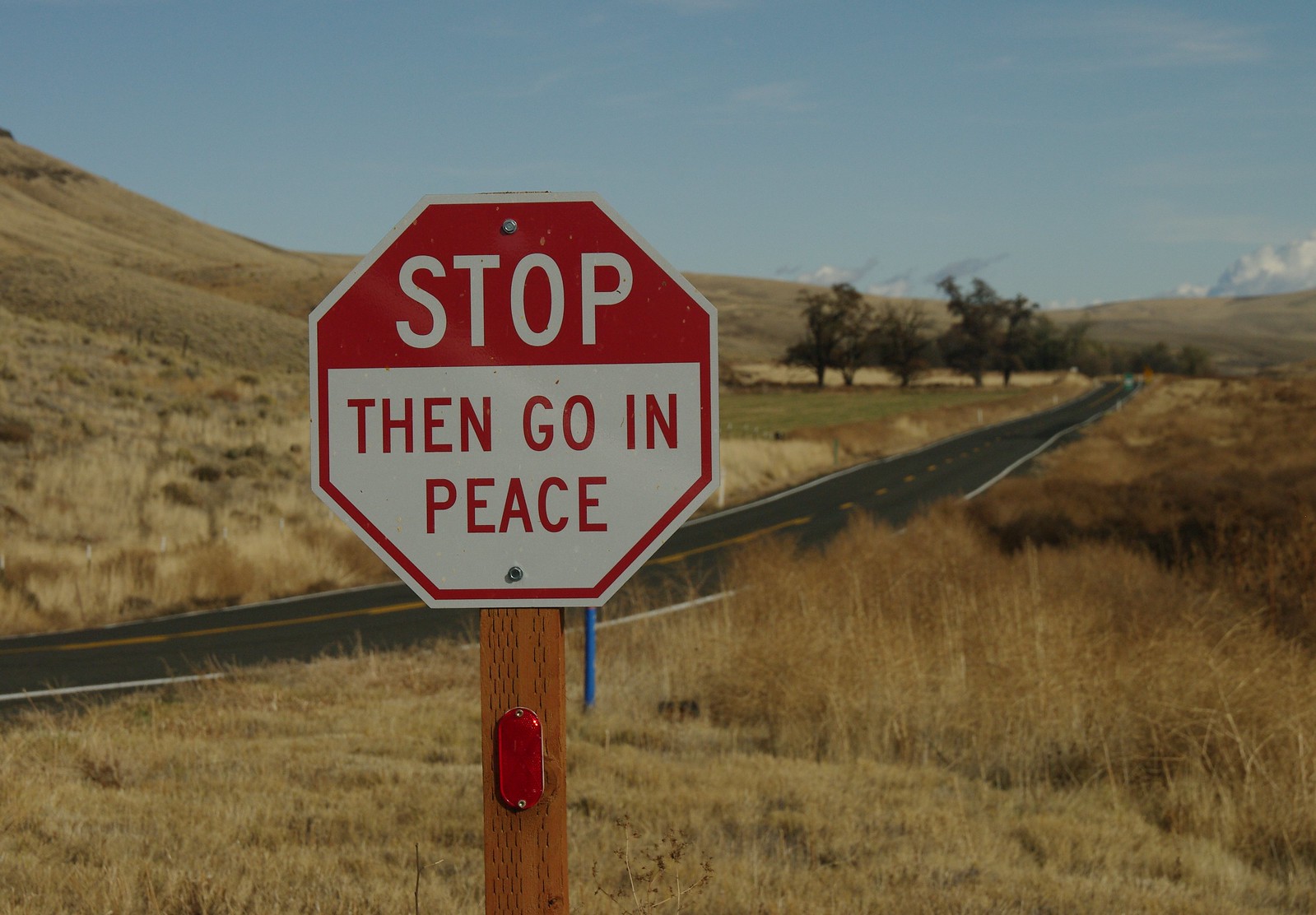In this outdoor daytime photograph, a distinct reddish-brown stop sign takes precedence in the foreground, standing out against a backdrop of rolling hills. The hills are cloaked in brown grasses, suggesting either the dryness of a late summer season or the barrenness left behind by winter. Sporadic trees dot the distant landscape, adding vertical interest to the otherwise undulating scenery. A freshly paved road slices through the hills, its smooth surface gleaming under the clear sky. The stop sign, an intentional variation with an additional message, reads, "Stop" at the top in white letters against a red background, typical of traditional stop signs. Below this, it bears a unique inscription: "Then go in peace." Mounted on a sturdy post, the sign also features a red reflector, ensuring it remains visible at night. The weather is impeccably clear, with not a single cloud marring the brilliant blue sky above.